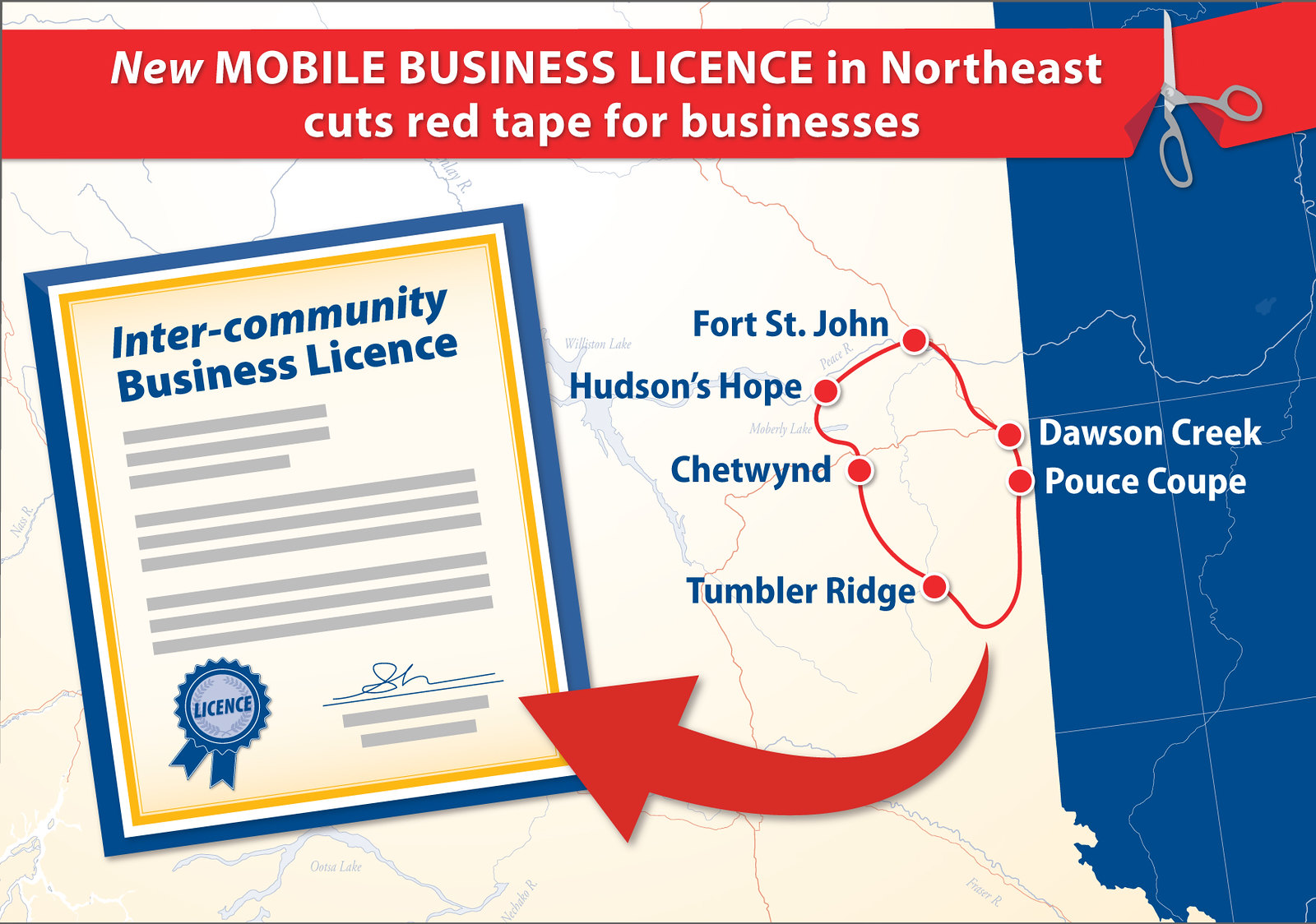This horizontally aligned rectangular image is a digital infographic centered on promoting a new mobile business license. It features a thin black border and a prominent red banner at the top with white text that reads "NEW MOBILE BUSINESS LICENSE" and "Northeast cuts red tape for businesses." The banner is symbolically being cut by gray scissors. 

The image's background is a map; the left and center sections have a light gray background interspersed with red and blue lines, representing roads, and narrow blue areas indicating lakes. In contrast, the right side of the image has a solid blue background with some white lines. 

Against the light gray background on the left side, a square framed with blue and gold borders contains a blue text header, "Inter-Community Business License," and placeholder horizontal gray bars, likely for additional text. Below this square is a blue ribbon that reads "License." 

A central feature of the image is a red line connecting several dots in a circular pattern. These dots represent different communities, labeled as Fort St. John, Hudson's Hope, Chetwynd, Tumbler Ridge, Dawson Creek, and Pouce Coupe. A large red arrow points from this circular arrangement towards the "Inter-Community Business License" square, emphasizing the connection between these locations and the new licensing initiative.